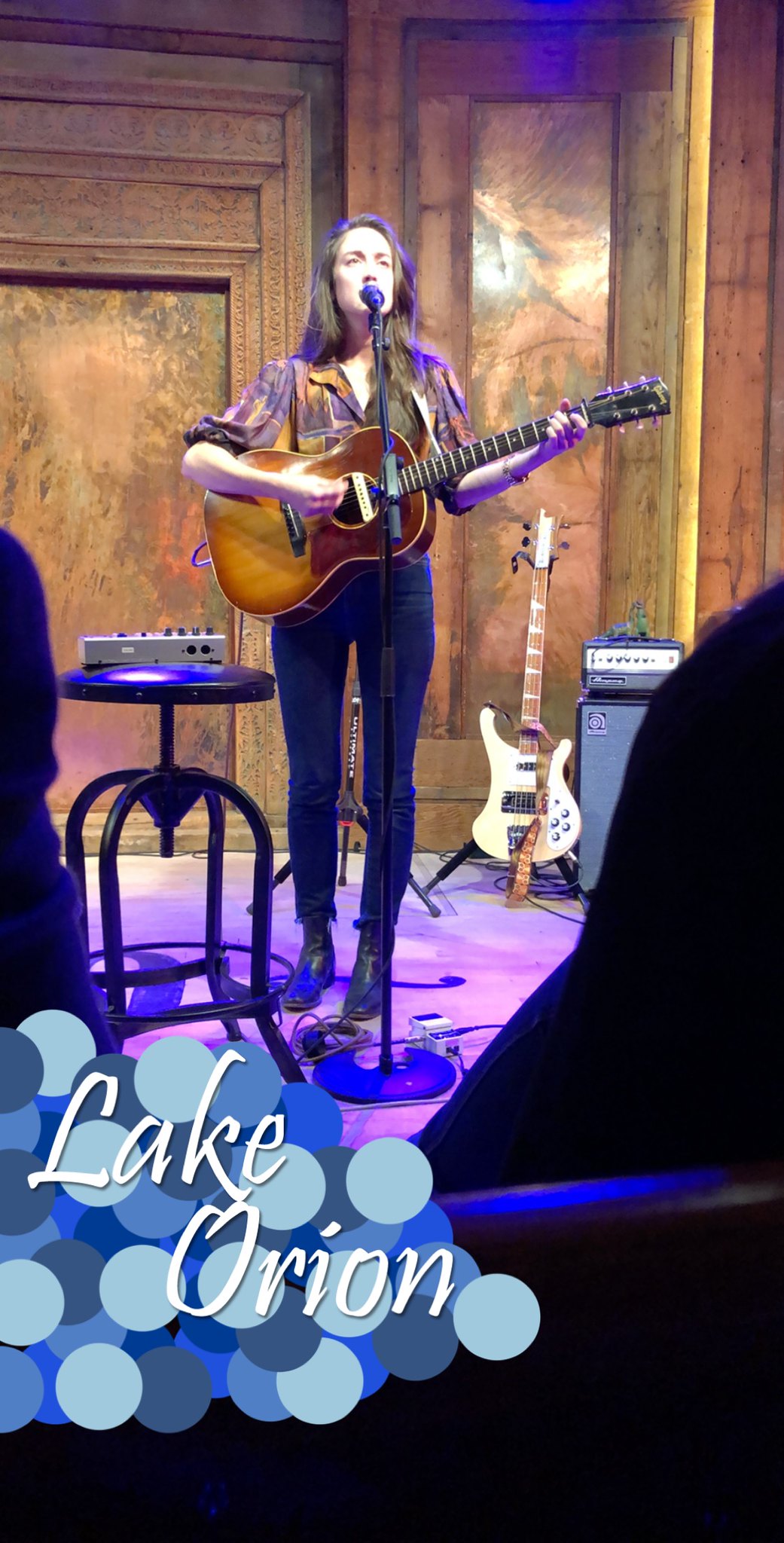This indoor photograph captures a young Caucasian female musician performing on a small stage. She has long, straight brown hair parted on the side, reaching past her shoulders. Dressed in a brown button-up blouse with the sleeves rolled up to the elbows, she pairs it with blue jeans and black boots. She is holding a brown acoustic guitar and is singing into a microphone on a tall stand. To her left, there's a stool with what appears to be an electrical board or a metal device on it. Behind her to the right, a lighter-colored electric guitar rests on a stand next to an amplifier. The backdrop consists of wooden frames and a brown wall. At the bottom of the image, an artistic overlay features overlapping blue circles with white text that reads "Lake Orion." The photo captures her in the center with the audience's shoulders framing her from both sides.